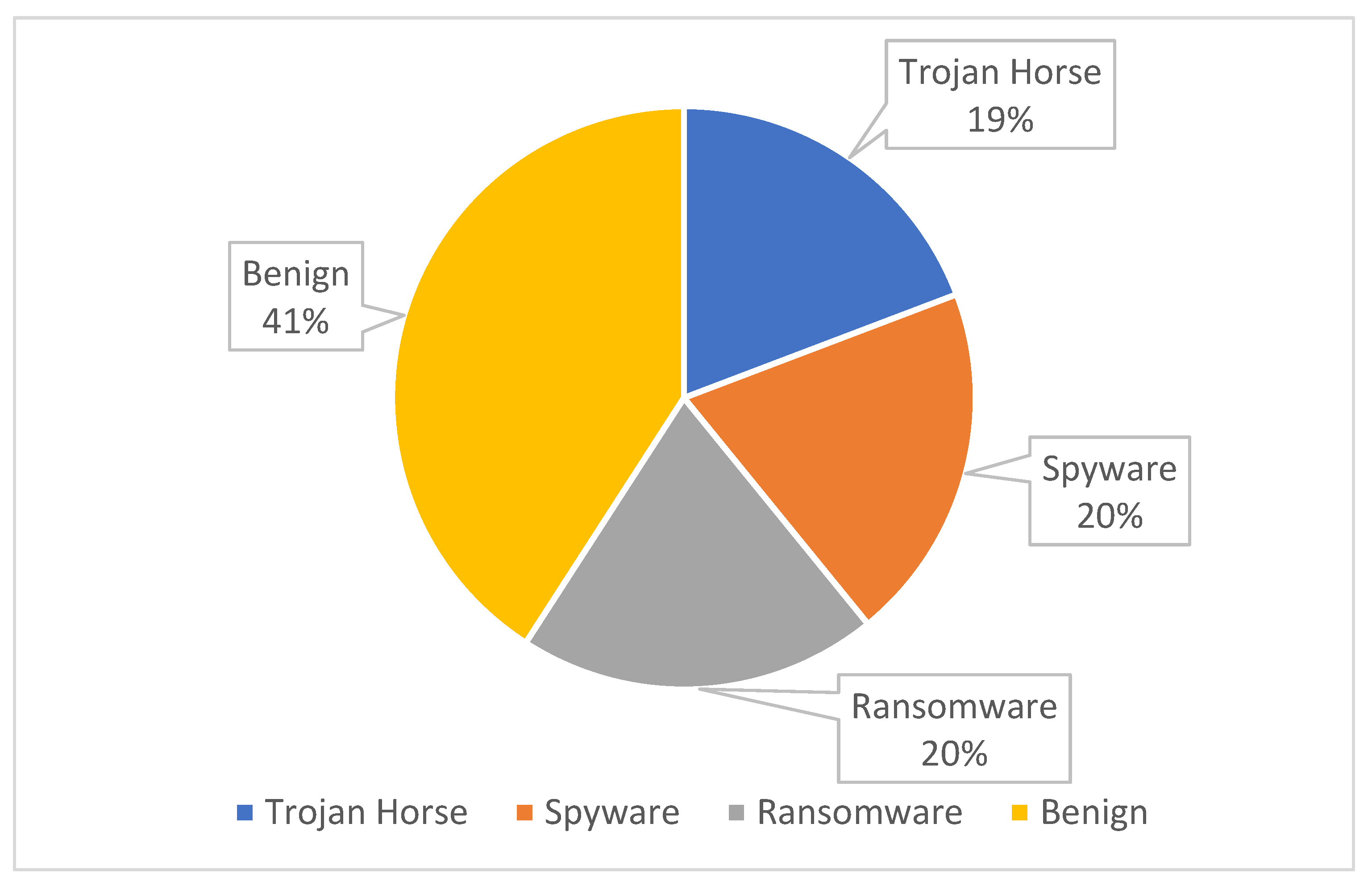The image is a detailed pie chart, likely sourced from a research article or journal. It features four segments, each differentiated by color and representing varying proportions of data. The colors used are yellow, blue, orange, and gray. The yellow segment occupies the largest portion of the chart at 41%, labeled "Benin" in black text. The blue segment, labeled "Trojan Horse," accounts for 19%. Both orange and gray segments each constitute 20% of the chart, with the orange labeled "Spyware" and the gray labeled "Ransomware." Additionally, at the bottom of the image, there is a legend with small colored squares corresponding to each category: a yellow square for Benin, blue for Trojan Horse, orange for Spyware, and gray for Ransomware. The pie chart is set against a white background, with each label pointing to its respective section on the chart.